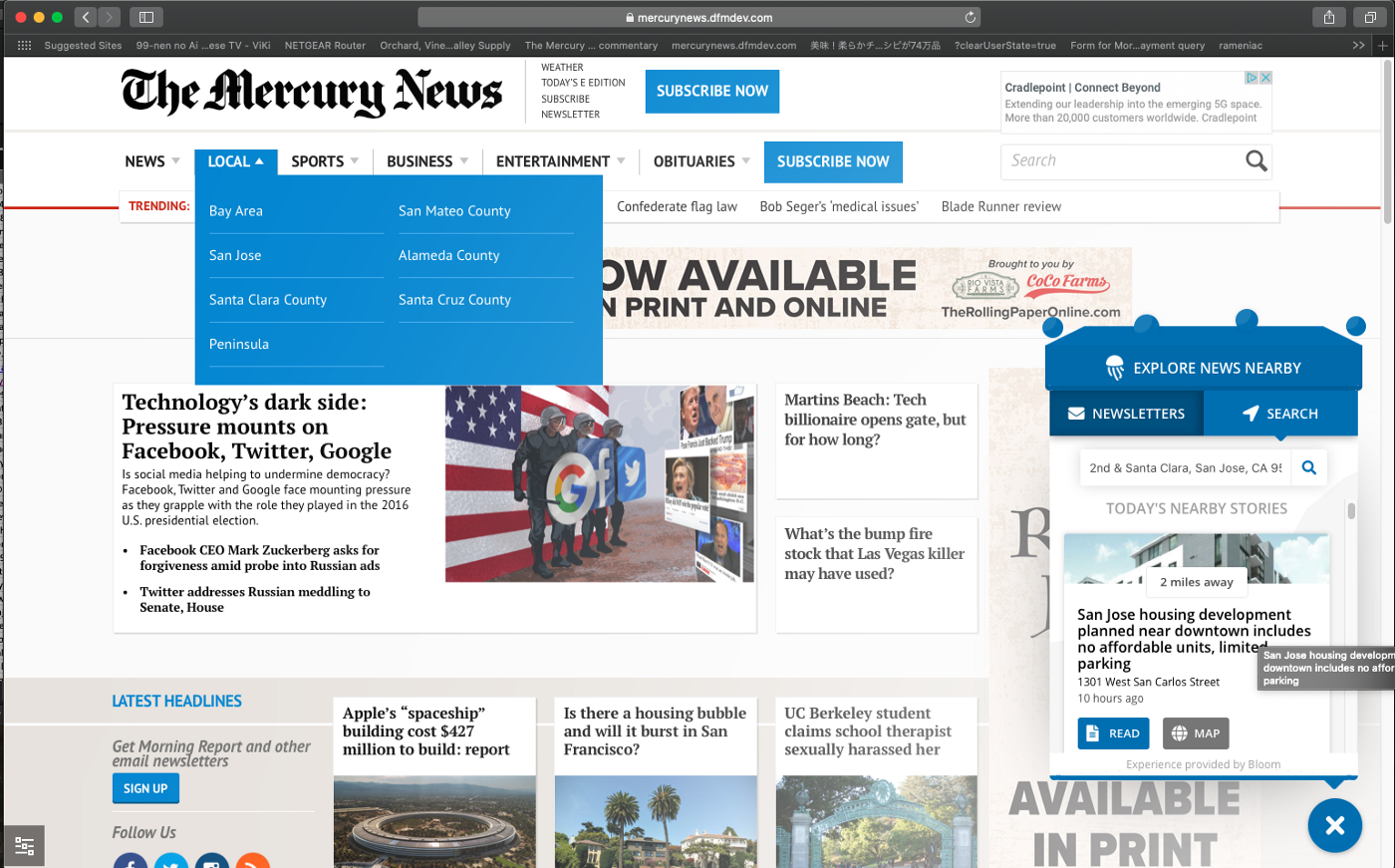A detailed screenshot of the Mercury News website showcases its comprehensive layout and featured content. On the far right side of the page, there is a prominent ad for Cradlepoint, emphasizing their expanding leadership in the emerging 5G market and highlighting their service to more than 20,000 customers worldwide. 

The Mercury News website offers a variety of options for readers, including sections for weather updates, today's edition, subscription services, and newsletters. Key interactive elements include prominently placed buttons such as "Subscribe Now" and drop-down menus that offer easy navigation to categories like news, local, sports, business, entertainment, and obituaries. 

In terms of content, featured articles cover diverse topics, including new legislation concerning the Confederate flag, Bob Seger's medical issues, and a review of the film Blade Runner. The screenshot captures the "Local" drop-down menu which, when selected, provides further options to drill down into regional news from Bay Area regions including San Jose, Santa Clara County, Peninsula, San Mateo County, Alameda County, and Santa Cruz County.